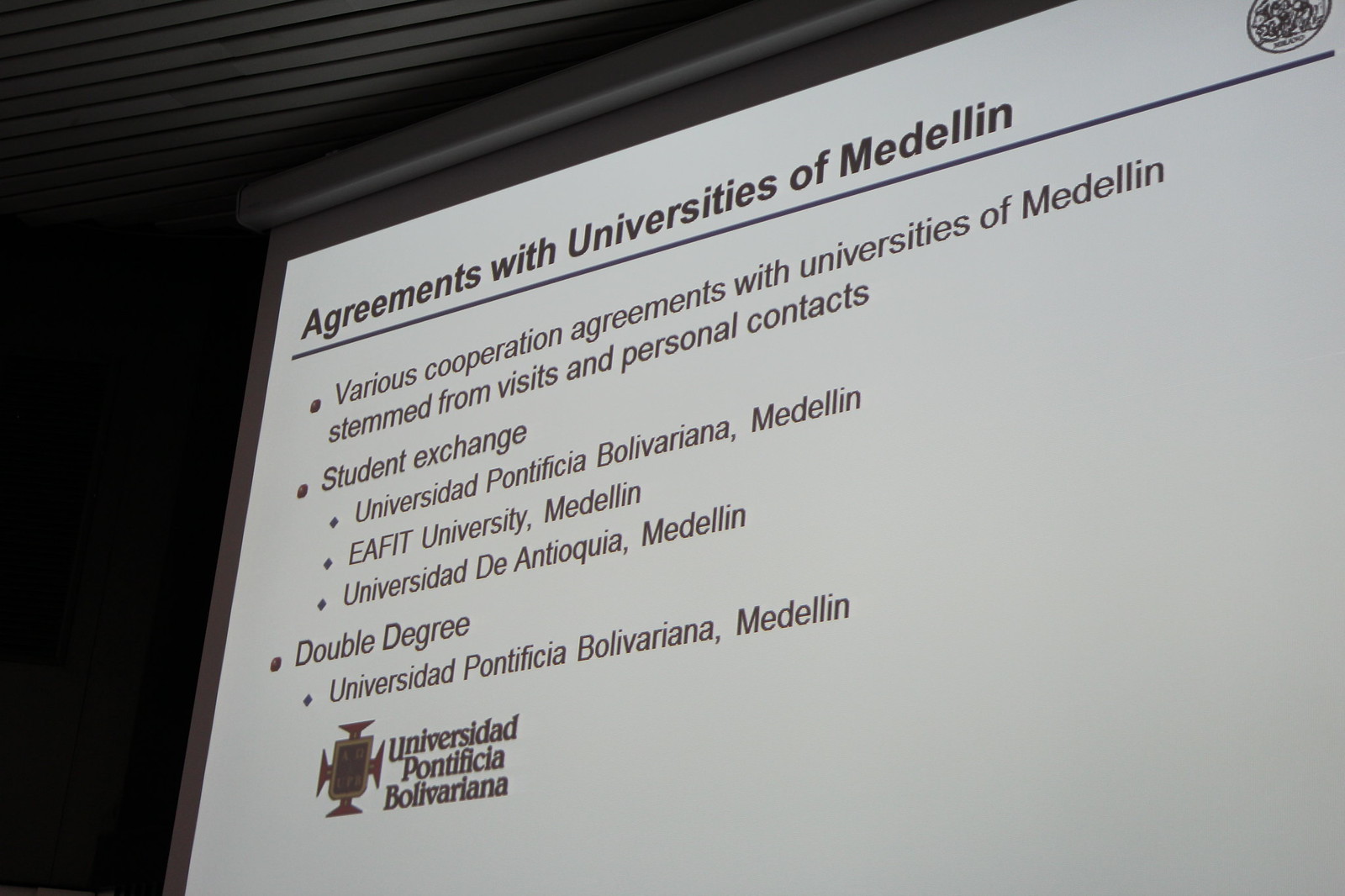This detailed photograph captures a classroom setting where a slide is being projected onto a screen. The screen displays black text against a white background, emphasizing "Agreements with Universities of Medellin." The text elaborates on various cooperation agreements with these universities, highlighting that they stemmed from visits and personal contacts. Designed to inform an audience, possibly students, about international collaborations, the slide also mentions student exchange programs and other partnerships. The image was taken from a lower angle, likely by someone sitting down, providing a clear view of the slide against a contrasting black wall, indicative of a formal presentation environment in a higher education institution.